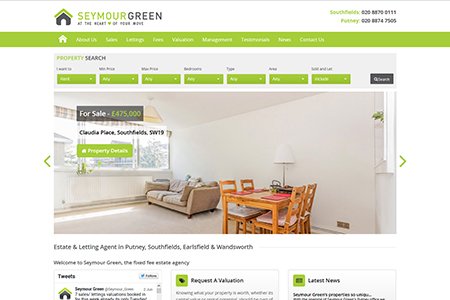This image is a screenshot of a real estate website named "Seymour Green," specializing in the selling and buying of houses in the UK. The screenshot appears zoomed out, making the font difficult to read due to its small size. On the top right corner, there is a contact number for reaching the agency.

The website features a property search functionality, with prices listed in pounds, indicating its UK base. Prominently displayed is a "For Sale" listing at £475,000 for a property in Claudia Place, Southfields. Below this listing, there is a button labeled "Property Details," which leads to more information about the house.

The image also includes a visual of a living room featuring a couch, lamp, and what appears to be a dining table. At the bottom of the page, there are sections dedicated to the latest news, options to request a property evaluation, and links to the agency's Twitter feed. Users can also find ways to contact agents and arrange property inspections.